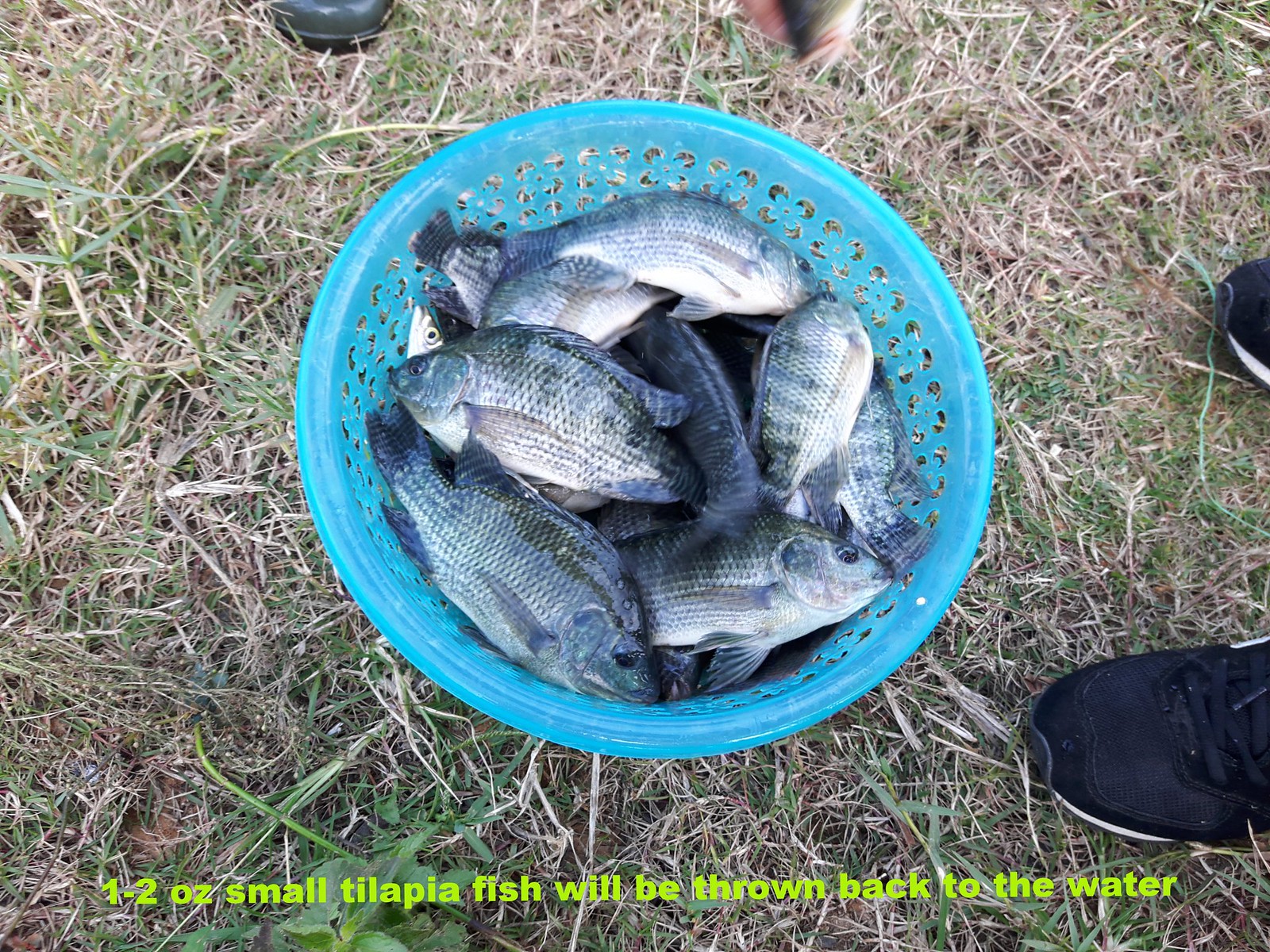A top-down view of a perforated, semi-transparent blue plastic bucket filled with small tilapia fish covered in vibrant silver and green scales, their distinctive boxy shapes making them easy to identify. The bucket, sitting on a patch of browned dead grass interspersed with occasional green blades, contains at least 15 tilapia, each around one to two ounces in weight. A caption in bright green text at the bottom of the image reads, "One to two OZ small tilapia fish will be thrown back to the water." In the scene, two pairs of shoes are visible: to the right, black tennis shoes with white accents, and at the top, the toes of black reflective boots, emphasizing the presence of people overseeing the fish.